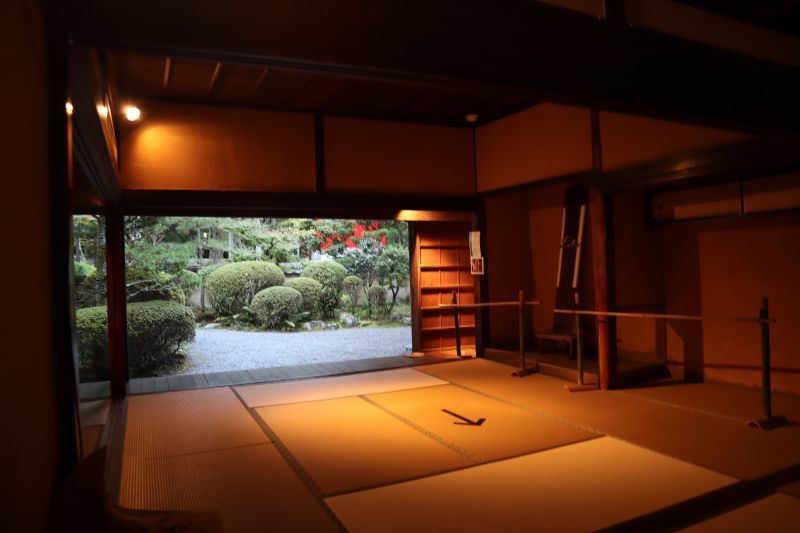The image showcases the dimly lit interior of a building, possibly a temple, constructed from dark brown wood that lines the walls and ceiling. The scene is illuminated by a single, warm, orange light in the top left-hand corner. The interior floor is covered with light brown mats, and a black arrow pointing towards the bottom right-hand corner adorns the center-right side of the floor. The right side of the image features a wall, while the left side has an area that appears to be either a mirror, window, or another doorway reflecting the outside. There is an opening in the wall towards the back left-hand side of the room. Outside, through the open doorway or wall, a gray stone pathway is bordered by meticulously trimmed topiary trees and green shrubs, with clusters of red plants visible in the background.